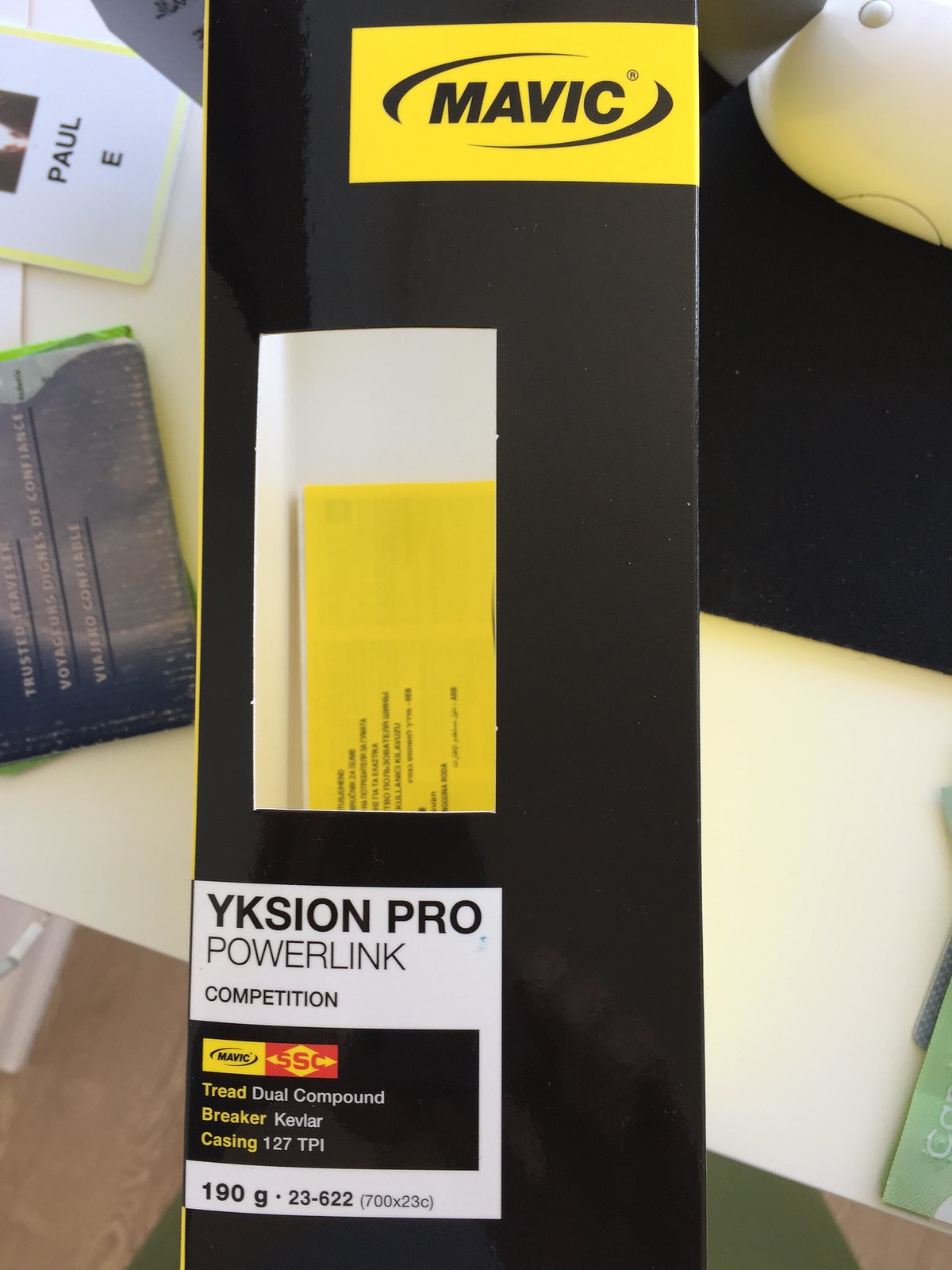This is a full-color image showcasing black Mavic packaging, prominently featuring a yellow rectangle with the Mavic logo at the top. The logo, in black text, is enclosed within a black circle on a yellow background. The box has a central viewport that reveals a yellow warranty information sheet inside, although the text on this sheet is unreadable. Near the bottom of the packaging, there is a prominent white rectangle containing detailed black text. It reads: "YKSION Pro PowerLink Competition." Below this, additional technical specifications are listed: "Tread Dual Compound, Breaker, Kevlar, Casing, 127 TPI, 190G, 23-622 (700X23C)." The backdrop for this photo is a cluttered desk featuring various items, including white and green papers, a name tag with "PAUL HEAT" written on it, and an old Apple mouse on a mouse pad.